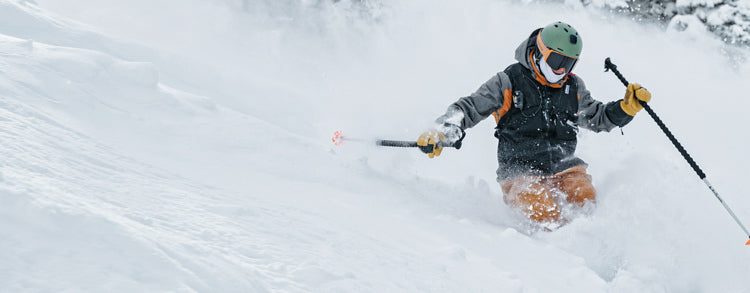The image captures an exhilarating winter scene on a snow-covered mountain, depicting a skier navigating down a steep slope enveloped in knee-deep powder. The photograph is bathed in white, with snow dominating the frame and creating a sense of motion as it is kicked up by the skier. In the background, faint outlines of snow-laden trees add depth to the scene, barely visible through the snowy haze. The skier is dressed in a stylish and functional outfit, consisting of an olive green helmet adorned with orange ski goggles, and a white ski mask covering their face for warmth. Their upper body is clad in a dark gray vest layered over a light gray and orange ski jacket with a hood. They sport yellow gloves and brownish pants, with ski poles that are black on the top half and white on the bottom, featuring orange baskets. The detailed and vibrant attire stands out against the wintry backdrop, highlighting the skier's motion and the thrill of the downhill descent.